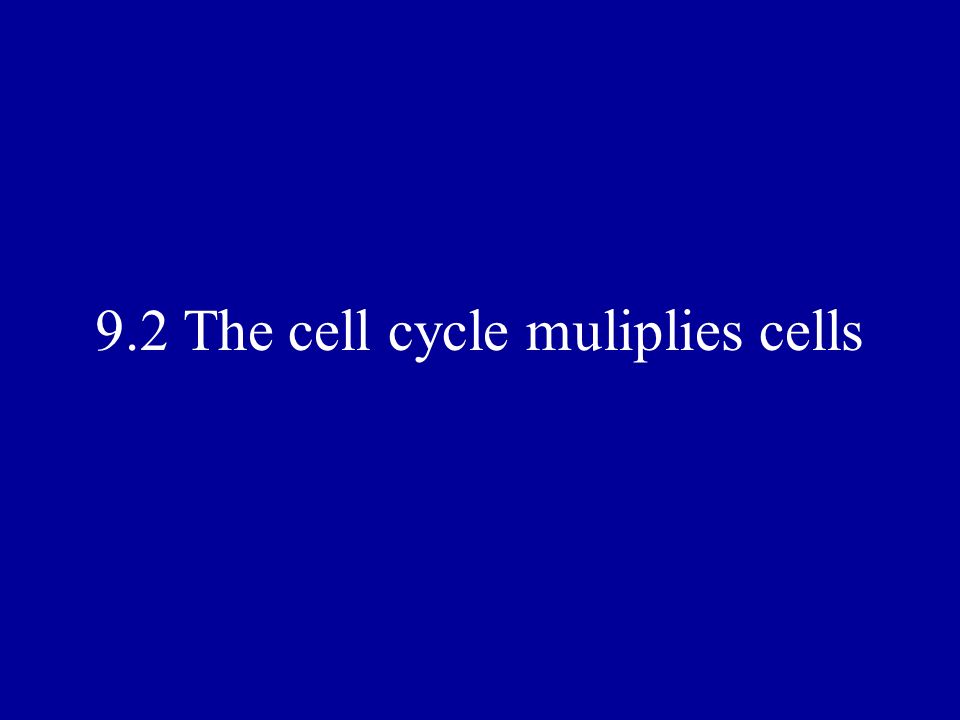This image features a vivid, solid blue background without any patterns or additional icons. Centered horizontally in white text are the numbers and words: "9.2 The cell cycle multiplies cells." The image appears to be a simple rectangular or square design, possibly part of a larger educational material like a book chapter or a section heading. Despite the incorrect spelling of "multiplies" as "m-u-l-i-p-l-i-e-s" in the third description, it illustrates the fundamental concept of cell cycle multiplication. The straightforward composition focuses solely on the blue background and white text, making the message clear and unembellished.